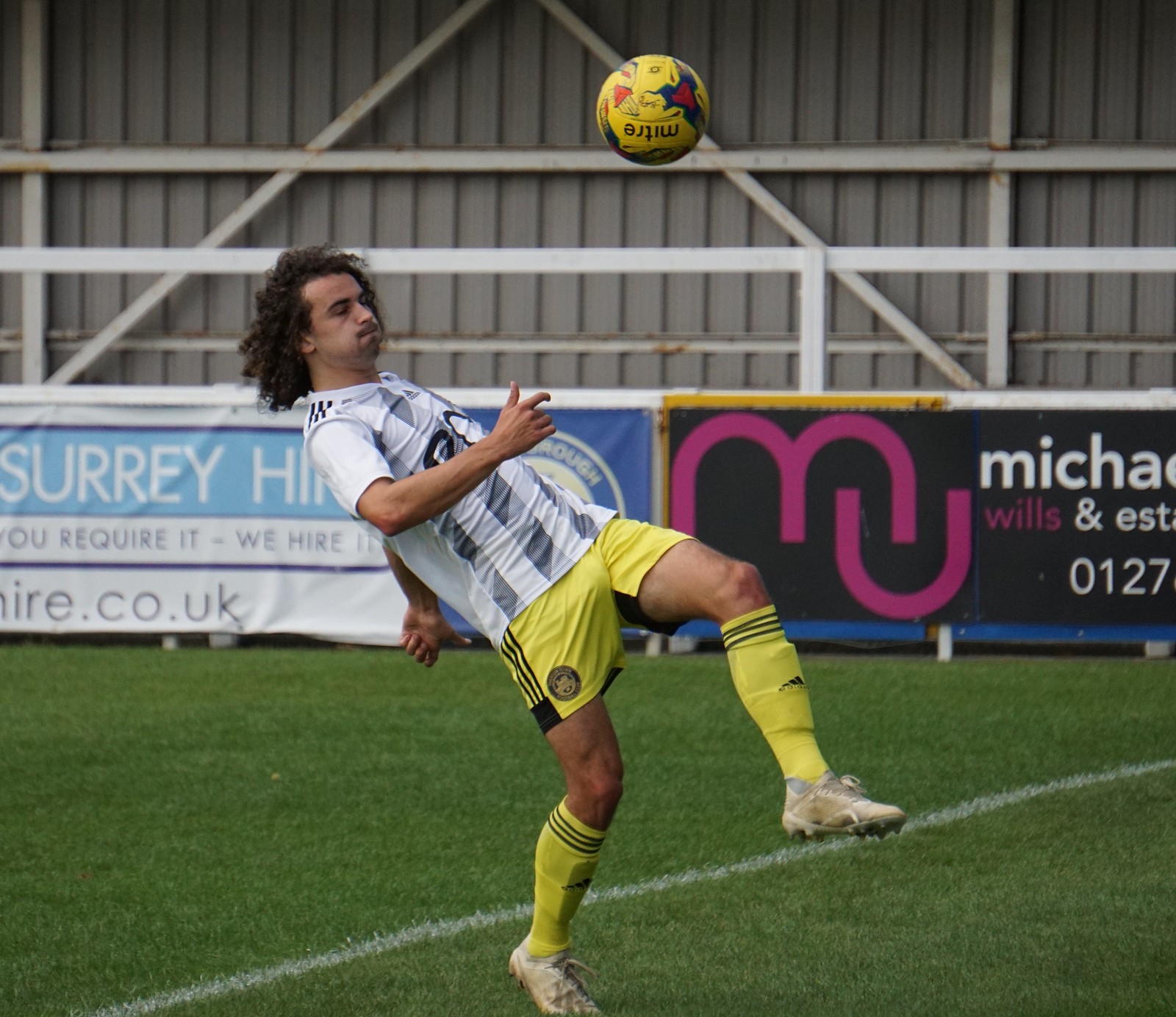In this detailed photograph, a single soccer player is captured mid-action on a green grass soccer field. He has light skin and long, dark, curly hair flowing down his back as he bends backward, balancing on his right foot with his left foot kicked high in the air. He is performing an acrobatic kick towards a yellow soccer ball, emblazoned with "MITRE" and featuring a black graphic design, which hovers several feet above him.

The player is clad in a white and gray vertically striped short-sleeve jersey, neon yellow shorts with black stripes along the sides, matching neon yellow socks with three black stripes at the top, and white soccer shoes with subtle brown details.

Behind him, a sponsorship banner stretches horizontally across the image. The banner includes a variety of text and colors, with some of the visible words being "Surrey Hill," "you require it, we hire it," and a partial website address "IRE.CO.UK." Another part of the banner has a black section with red lettering stating "M-U" and "Michael" in white underneath. The backdrop further includes a dark gray metal wall with rust-streaked white metal framing, adding an industrial feel to the scene. The overall setting is outdoors, capturing the dynamic moment of a soccer game.